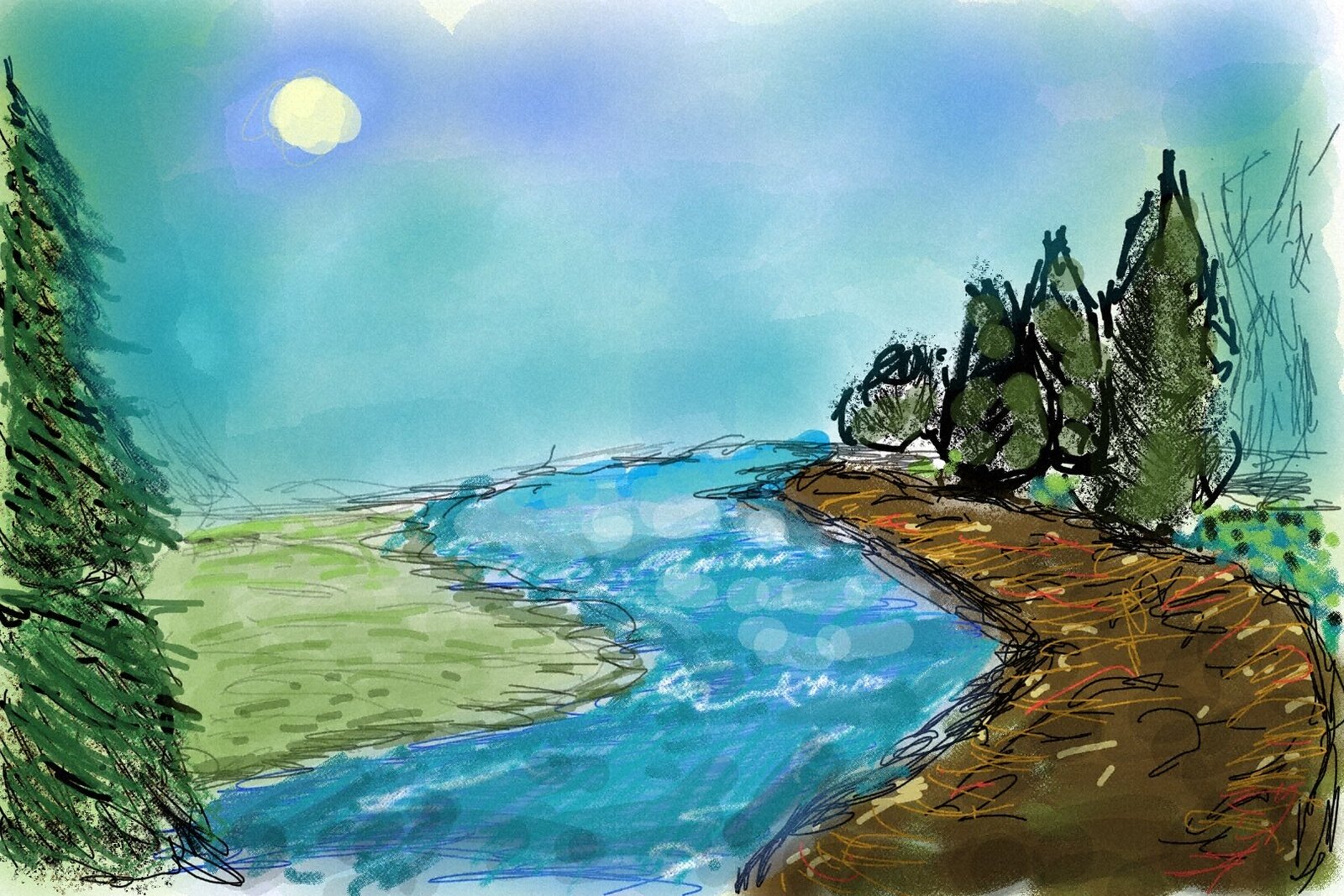The image depicts a scenic landscape rendered in a somewhat crude, watercolor style. The backdrop features a clear blue sky with a round, white sun situated in the top-left corner. On the left side of the image, a prominent cedar tree stands alongside a light green grassy patch, which transitions into a blue, gently rippling stream. The stream meanders upward, lined by a brownish riverbank displaying squiggly lines in shades of orange and yellow. On the right side of the stream, additional cedar trees rise above the earthy riverbank, contrasting with a broader expanse of green grass. The scene captures a harmonious interplay of natural elements, showcasing the tranquil beauty of a forested river landscape.